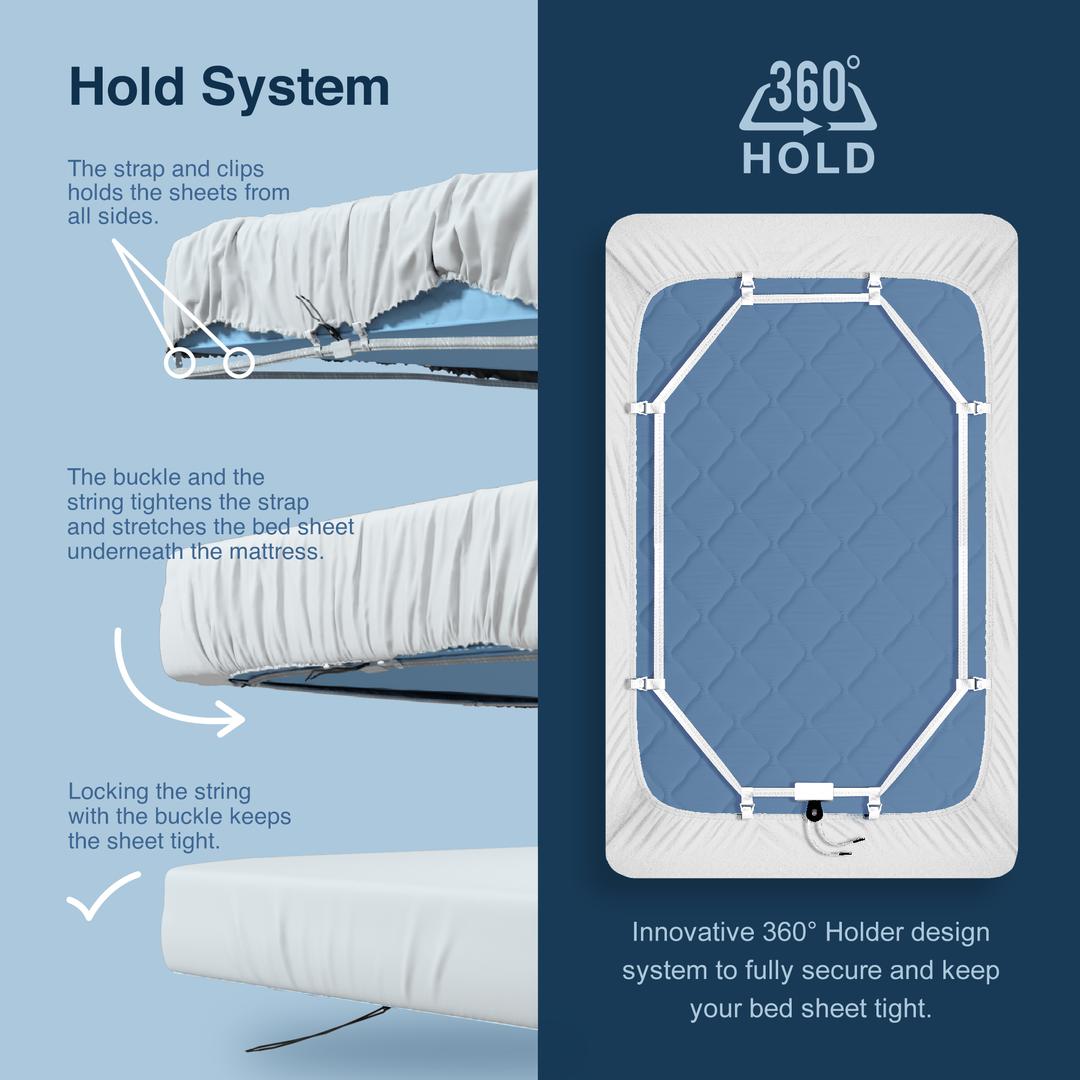The image appears to be a part of an advertisement for a mattress cover, showcasing a system designed to keep fitted sheets tightly secured. The left side of the image, set against a light blue background, demonstrates the "Hold System" in a three-step visual guide. The first photograph shows a bare mattress with a caption explaining how the straps and clips hold the sheets from all sides. The second image illustrates the buckle and string mechanism that tightens the strap and stretches the sheet beneath the mattress. The final picture on the left depicts the fully secured fitted sheet with a note that locking the string with the buckle keeps the sheet tight.

On the right side, the background shifts to dark blue and prominently displays the "360° Hold" system, described as an innovative design to fully secure and keep the bed sheet tight. This side features a detailed view of the underside of a mattress, highlighting the straps and clips in action along the edges. The accompanying text emphasizes the 360° holder design, which mimics a suspender mechanism, attaching the fitted sheet to the mattress from all sides to ensure it remains taut and in place. The entire layout is neatly divided with visual aids and textual descriptions, cohesively demonstrating the functionality and benefits of the 360° Hold system to potential customers.